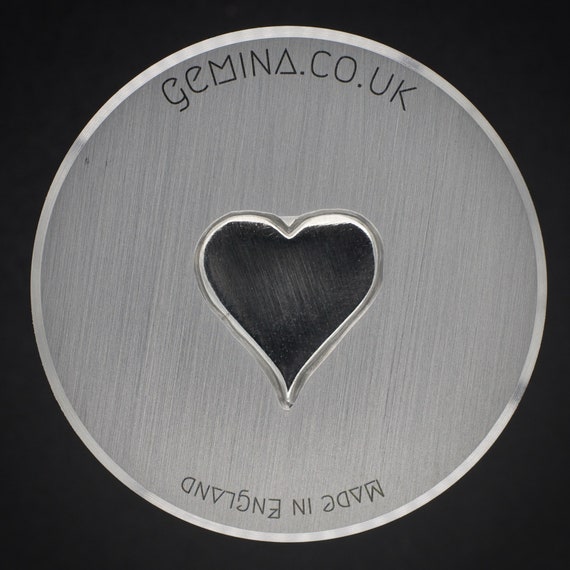This photograph features a circular, coin-shaped charm composed of brushed silver, displayed against a black background. Central to the charm is a heart shape, filled with a dark black color, and edged with a white border. Surrounding the heart, the charm itself has a white edge, followed by a darker gray outer border. The silver coin has detailed inscriptions; at the top, the text reads "Jemina.co.uk," with unique typographic features such as the 'A' being represented as a triangle and the 'M' having a line connecting the two vertical lines. Along the bottom edge, the phrase "Made in England" is inscribed upside down, employing similar typographic characteristics for the letters 'A' and 'M'. The photo is shot from a top-down perspective, ensuring an even spacing around the charm, highlighting the distinct features and the textured quality of the materials used.